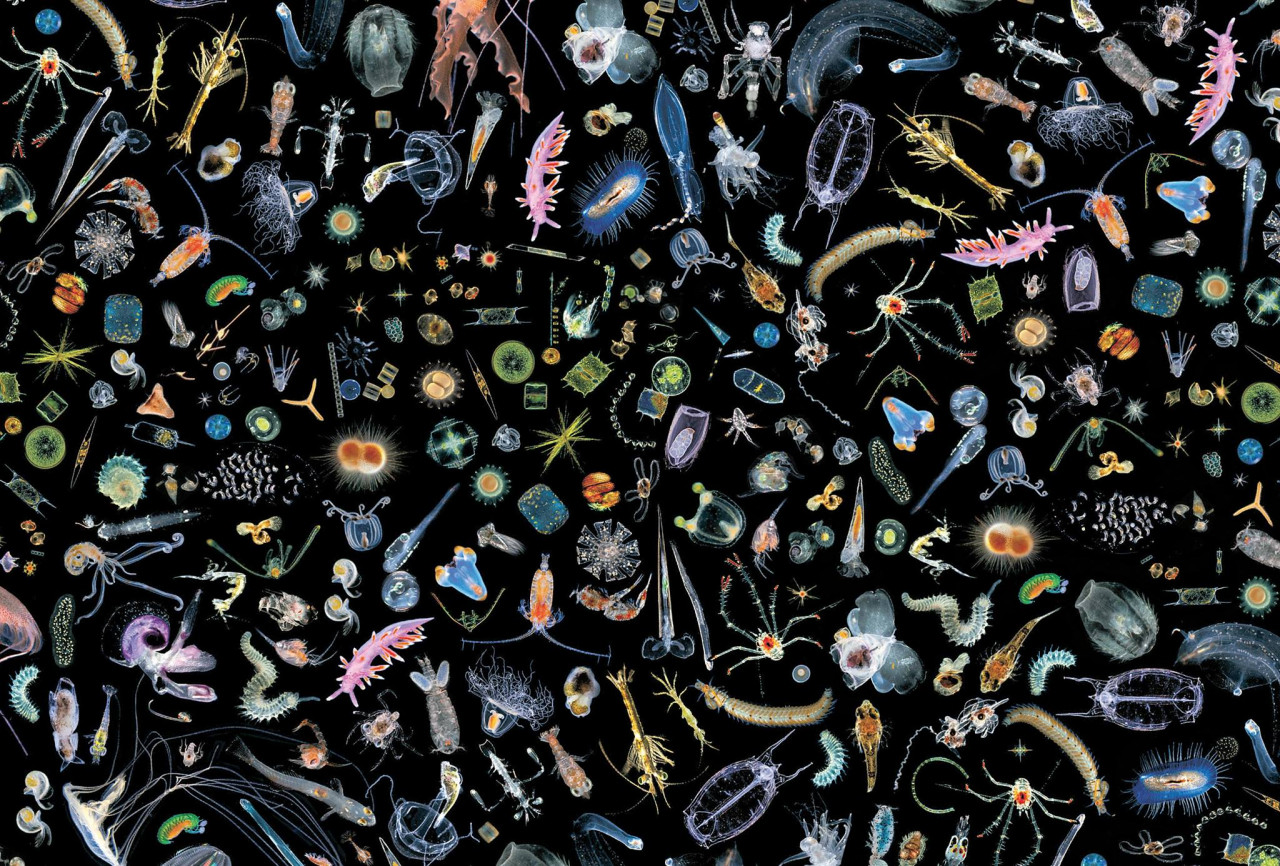This intricate drawing showcases an array of approximately one hundred or more small creatures against a stark black background. The diverse creatures exhibit a variety of forms and colors, some reminiscent of sea animals or microscopic beings. Notable entities include several pink-bodied organisms adorned with spiny protrusions, primarily clustered in the scene. An orange creature with prominent white features and two antennae stands out in the top left corner. The lower right hosts a group of goldfish-like figures, while central areas are populated with jellyfish, starfish, and multiple forms of worms—ranging from brown and yellow to greenish-brown and green. Other notable shapes include star-like forms, spider-like entities, green globular figures evoking sea urchins, clear-bodied organisms with white internal masses, and a peculiar orange being resembling a neon cockroach. Despite the diversity and repetition among the critters, the image remains void of any text, offering only a visual tableau of imagined life forms in a meticulously crowded composition.